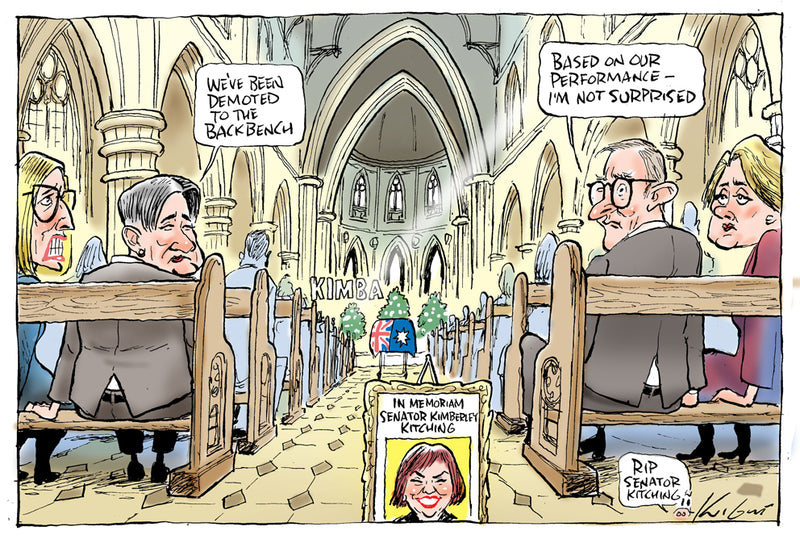In this detailed, full-color political cartoon, the scene is set inside a large church, depicted with arches and wooden pews lining both sides, creating an aisle down the middle. Centered near the back, a coffin draped in a flag—divided into blue with a star on the right and red and white crosses on the left—suggests a former British colony, though the specific nation is unclear. Flanking the coffin are three green plants and a flag, adding a poignant touch to the setting. Above the coffin, the word "Kimba" is visible.

Near the bottom center of the cartoon, a plaque inscribed "In Memoriam, Senator Kimberly Kitching" accompanies a smiling photograph of the late senator. In the lower right corner, beneath the back pew, a thought bubble reads "R.I.P. Senator Kitching," adjacent to a black signature marking the artist's name.

The cartoon's primary focus draws attention to four individuals seated at the back pews of the church, split into pairs on either side of the aisle. On the left, a woman with blonde hair and large black glasses, dressed in something blue, converses with a gray-haired man in a gray suit. Above them, a speech bubble reads, "We've been demoted to the back bench." On the right, a short-haired blonde woman in purple and a white-haired man, also in a gray suit with large black glasses, respond with a speech bubble saying, "Based on our performance, I'm not surprised." The cartoon's somber setting and the dialogue attempt to mix humor with the solemnity of the memorial, hinting at a critique of political status and performance.